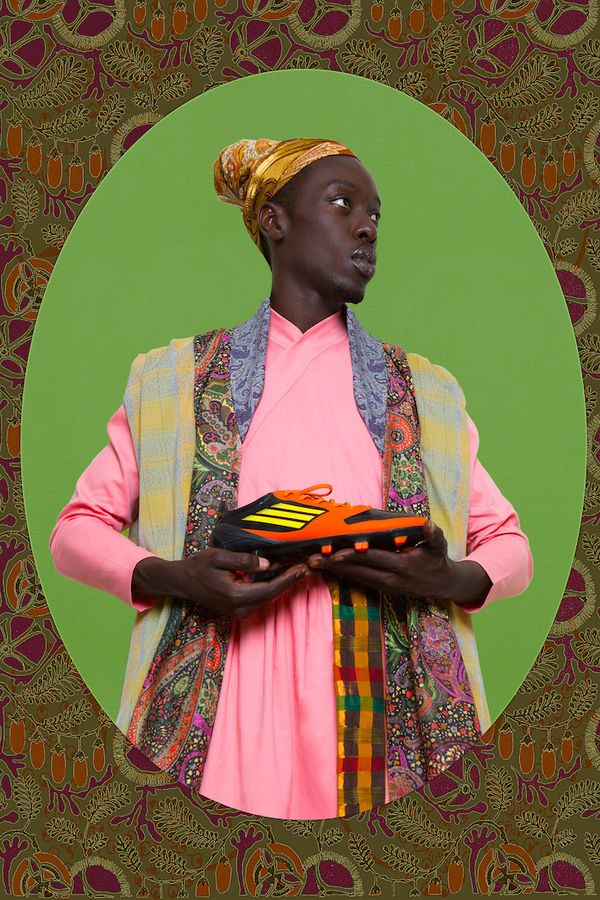This composite image features an African or African American woman with deep black skin, captured within an oval shaded green. The woman, adorned in a vibrant attire, has her head turned to her left, showcasing a serious expression, while her body faces forward. Her head is wrapped in a golden yellow scarf styled like a tight turban, covering a possible hair bun. She wears a striking bright pink dress with long sleeves and is draped in multiple scarves. The innermost scarf is gray with yellow stripes, the next one is a brilliantly designed paisley in pinks, greens, purples, and whites, and the outermost is a greenish-yellow muted tone with horizontal stripes. The woman holds an orange athletic shoe with cleats in her hands, marking its distinctive three yellow stripes and black details. The background of the image continues the paisley theme, presented in varying shades of green, gray, and pink, complementing the overall vibrant yet serious tone of the photograph.